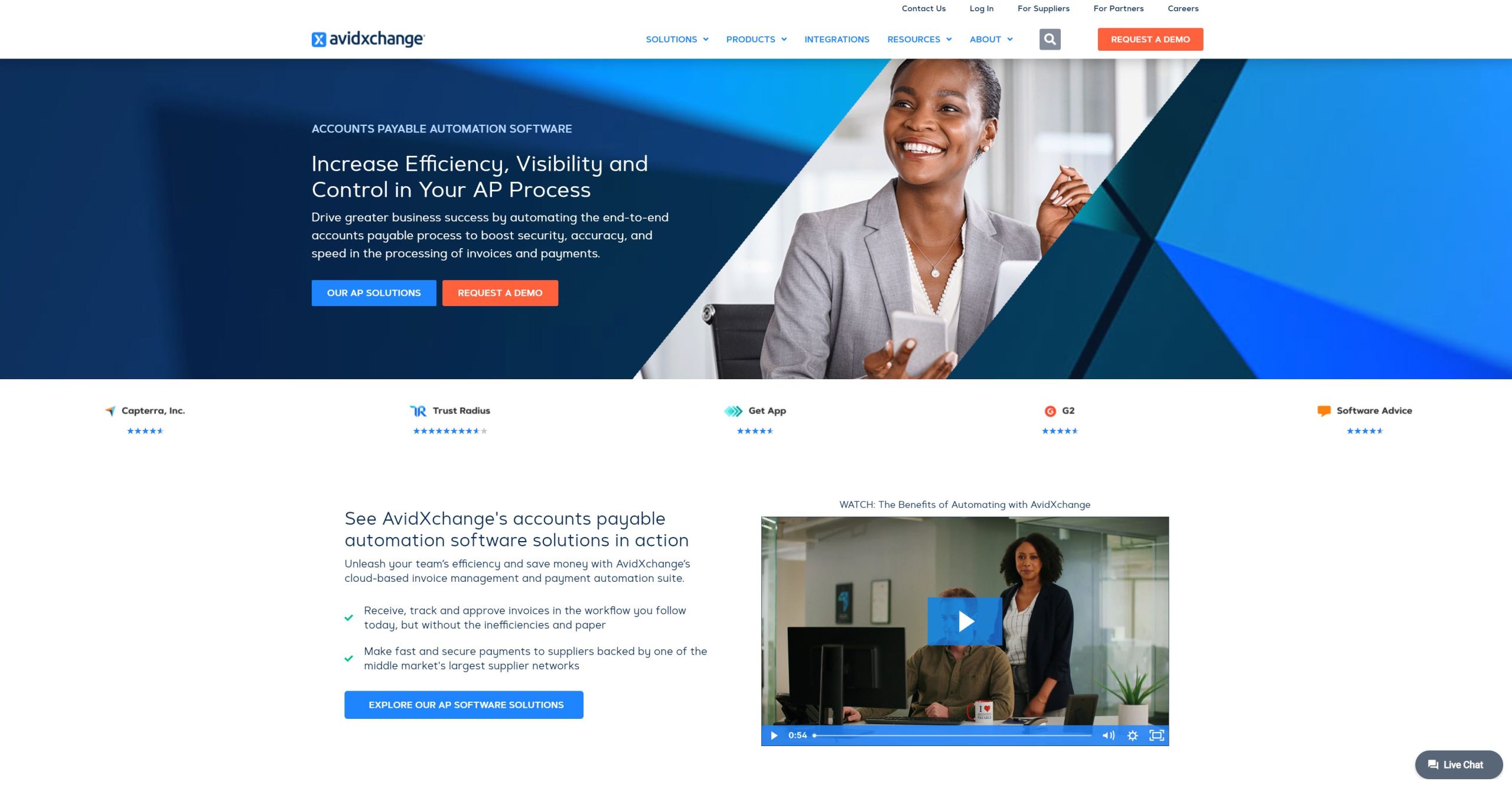This detailed screenshot captures the homepage of the Avid Exchange website, displayed on a computer or laptop. The navigation menu on the right includes sections for "Solutions," "Products," "Integrations," "Resources," and "About." There are multiple action buttons such as "Contact Us," "Login for Suppliers," "Login for Partners," and "Careers." Additionally, an eye-catching orange "Request a Demo" button is prominently featured.

Dominating the banner is an image of a smiling Black woman, who is elegantly dressed in a gray suit, white shirt, and white necklace. She holds a white phone and sits comfortably in a black chair, positioned in front of a white computer. The background of the banner employs various shades of blue, lending a professional and serene atmosphere.

Adjacent to the woman's image is informative text about the website, highlighted in the same blue tones. The lower left section of the banner page includes a paragraph elaborating on the website's offerings. Below this text, there is a paused 54-second video, titled "Watch the Benefits of Automating with Avid Exchange." The video thumbnail depicts two individuals: a man seated at a computer and a Black woman standing behind him, looking down. The scene is set with a coffee cup on the table and a plant in a white planter, adding a touch of warmth and reality to the workspace setting.